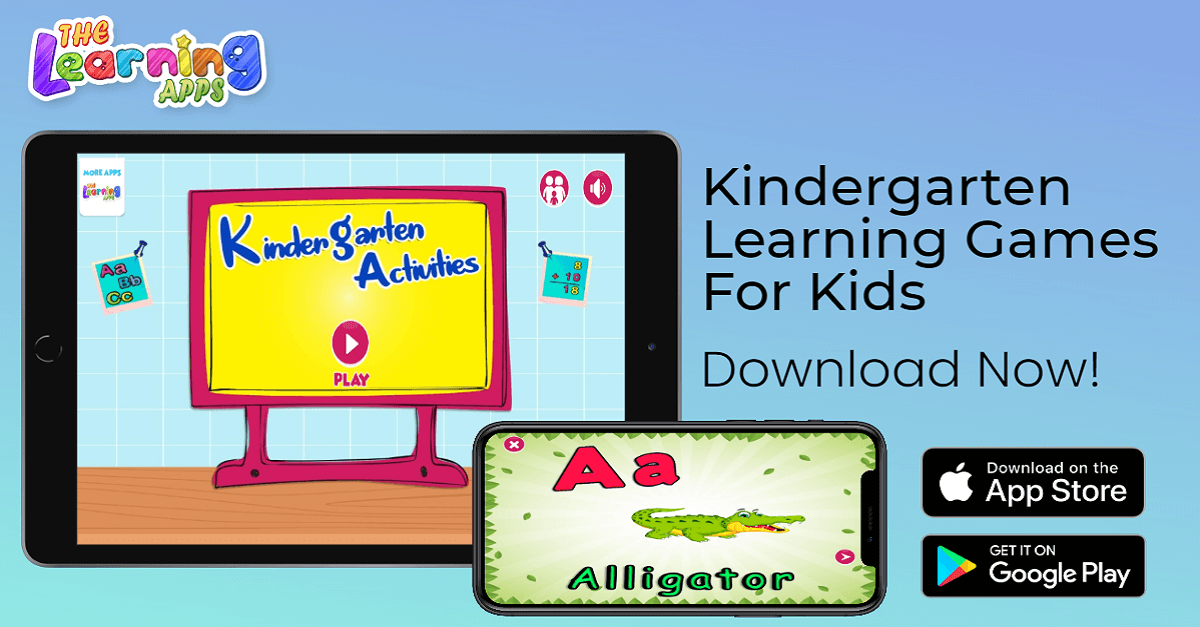The image features a dreamy ombre background that transitions from periwinkle at the top to a lighter sea breeze color towards the bottom. On the top left corner, the word "Dove" appears in orange with a red outline accentuated by a white border. Beneath this, the word "Learning" is displayed in a playful array of colors: purple, green, red, blue, pink, yellow, orange, and blue, each letter outlined in white. Below "Learning," the word "Apps" stands out in green with a white outline.

In the center of the image, there is a black tablet showcasing an app description. The app title, "Kindergarten Activities," is in blue, outlined in white, set against a yellow chalkboard background. Next to the tablet is a black smartphone with a green screen displaying an uppercase "A" and a lowercase "a" in red, next to a green alligator. The area around the alligator is yellow, and beneath it, "Alligator" is written in green.

On the right side of the image, a bold, black text reads, "Kindergarten Learning Games for Kids. Download Now!" Below this call to action, there are two download buttons. The first black rectangle features a white apple icon with the text "Download on the App Store," and the second black rectangle has the Google Play logo with the text "Get it on Google Play."